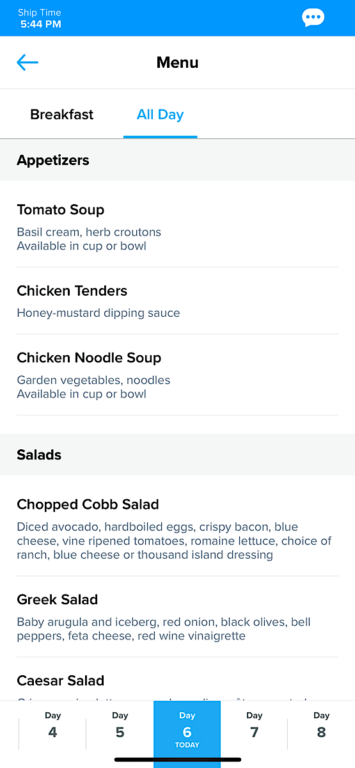This image is a screenshot of someone’s phone at 5:44 p.m. The top of the screen features a blue border, with the time displayed on the upper left and a word bubble with three dots on the upper right. Below this, there is the word "menu," followed by tabs labeled "Breakfast" and "All Day," with the "All Day" tab highlighted in blue and underlined.

The menu starts with the title "Appetizers," and includes three options: 
1. Tomato Soup - described as having basil, cream, herbs, and croutons, available in a cup or bowl.
2. Chicken Tenders - served with honey mustard dipping sauce.
3. Chicken Noodle Soup - featuring garden vegetables and noodles, available in a cup or bowl.

Following appetizers, the next section of the menu lists "Salads," providing three choices:
1. Chopped Cobb Salad - includes diced avocado, hard-boiled eggs, crispy bacon, blue cheese, vine-ripened tomatoes, and romaine lettuce, with a choice of ranch, blue cheese, or thousand island dressing.
2. Greek Salad - features baby arugula and iceberg lettuce, red onion, black olives, bell peppers, feta cheese, and red wine vinaigrette.
3. Caesar Salad - listed without a detailed description.

At the bottom of the screen, there are tabs labeled "Day 4," "Day 5," "Day 6," "Day 7," and "Day 8," with "Day 6" highlighted in blue.